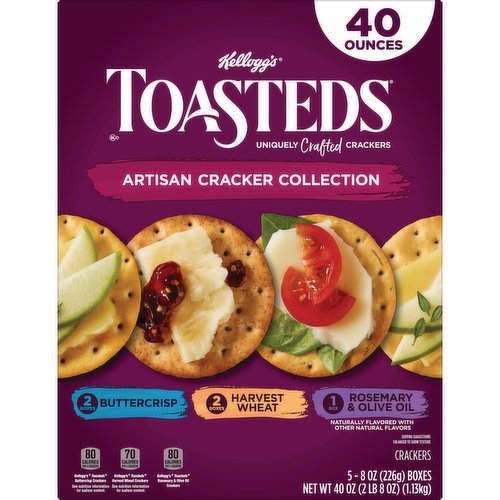This image depicts the exterior of a food box for Kellogg's Toasteds Uniquely Crafted Crackers. The rectangular box has a rich plum-colored background. At the top of the box, a white semicircle prominently displays "40 ounces" in plum-colored text. The upper third of the packaging features the brand name "Kellogg's" in white, above the product name "Toasteds" in large white font. Beneath this, the phrase "Uniquely Crafted Crackers" is also displayed in white.

A lighter plum-colored brushstroke carries the text "Artisan Cracker Collection" in white capital letters further down on the package. Centrally, the box showcases a horizontal row of four round crackers with various toppings that include combinations of fruits, cheese, tomatoes, lettuce, and spreads. Each cracker is labeled with different flavors: Butter Crisp, Harvest Wheat, and Rosemary Olive Oil, indicating variety in the package contents.

At the bottom of the box, it informs the customer that there are five 8-ounce boxes inside, making the net weight a total of 40 ounces (2 pounds, 8 ounces).